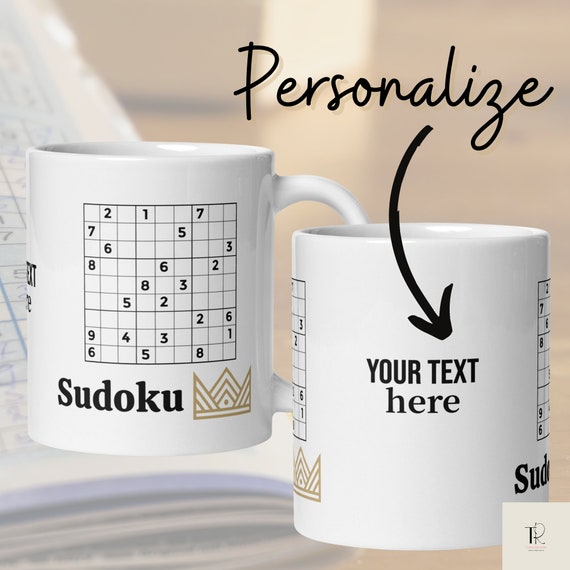This advertisement showcases two personalized coffee mugs from different angles against a blurred tan background featuring a Sudoku puzzle book. The mug on the left displays a standard Sudoku board with some numbers filled in, and below it, the word "Sudoku" is inscribed in bold text with a golden, crown-shaped design. The right mug shows a blank area labeled "Your Text Here," with the word "Personalize" written in cursive above it accompanied by an arrow pointing to the customizable text. In the bottom right corner of the image, the company initials "TR" are printed in a small, tan square. The setting suggests a customizable product sold through platforms like Etsy.